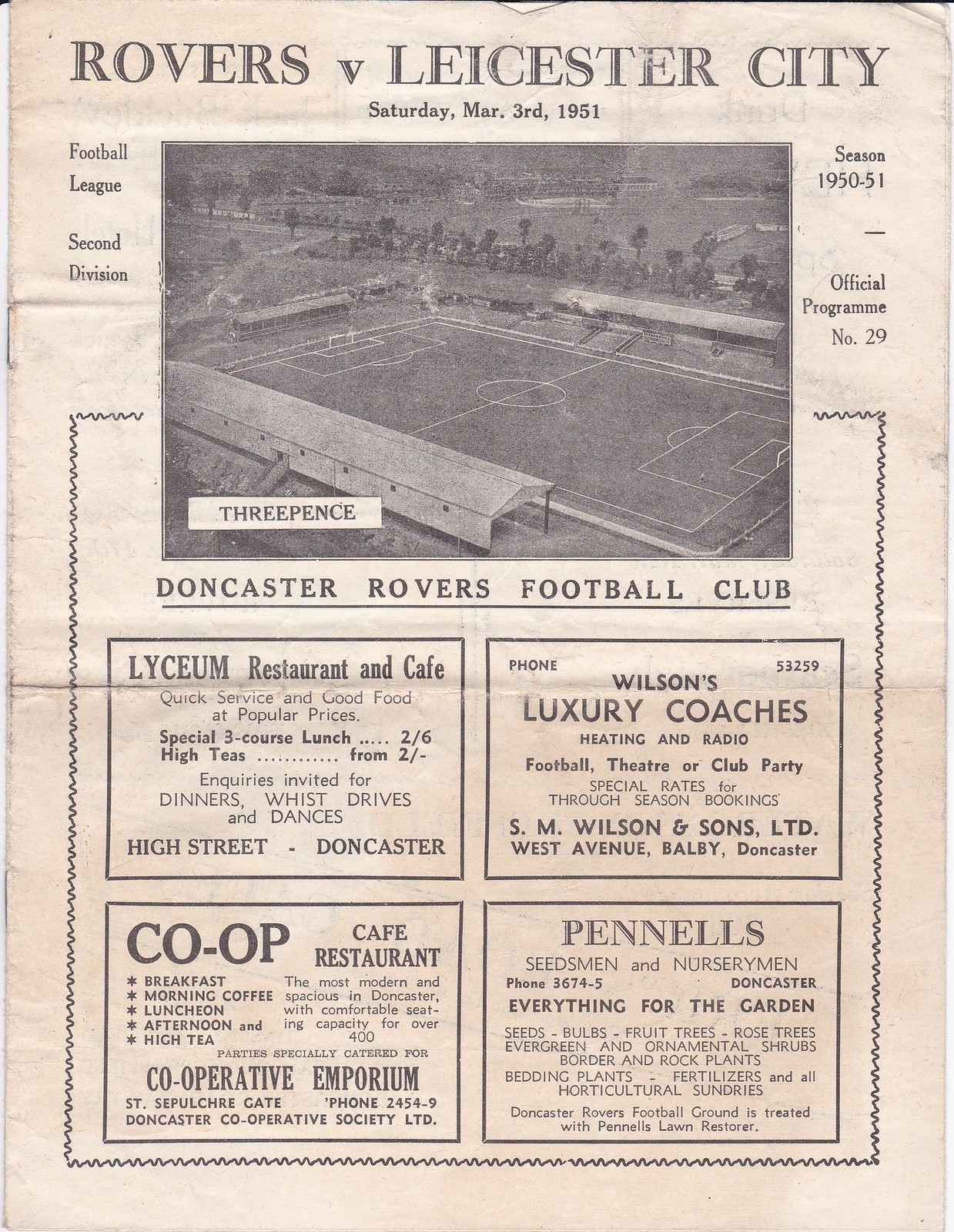This detailed caption integrates and cleans up the descriptions provided, focusing on shared and repeated elements while adding coherence and detail:

This image depicts an aged, yellowed page from an official soccer club program for the Doncaster Rovers Football Club, dated Saturday, March 3, 1951. The heading reads "Rovers vs. Leicester City" and details the match as part of the 1950-51 Football League 2nd Division season, specifically program number 29, priced at 3 pence. At the center of the page is a black-and-white aerial photo of a soccer field, labeled underneath with "Doncaster Rovers Football Club." Surrounding the image are four rectangular advertisements. The top-left ad promotes the Lyceum Restaurant and Cafe, highlighting quick service, good food at popular prices, and special 3-course lunches. Adjacent to it, the top-right ad advertises Wilson's Luxury Coaches, complete with phone number 53259 and amenities like heating and radio for football, theatre, or club parties, with special rates available for through-season bookings. In the bottom-left corner, the Co-op Cafe-Restaurant invites patrons to experience their modern and spacious establishment on St. Sepulchre Gate, known for accommodating over 400 guests and providing meals throughout the day, with a contact number of 2454-9. Lastly, the bottom-right ad from Pinell's Seedsmen and Nurserymen offers an extensive range of gardening supplies and services, including seeds, bulbs, and lawn restorer, listing their contact number as 3674-5. The page blends the vintage allure of old newspapers with a functional program layout.